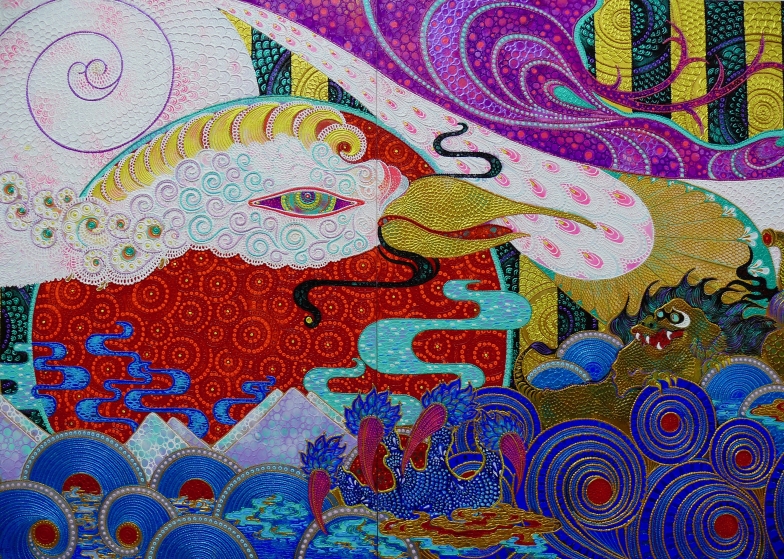This intricate, abstract artwork features a vibrant amalgamation of various elements and colors, creating a visually stimulating experience. At the center, a gold duck bill, adorned with a long, wavy Fu Manchu mustache, captures attention, radiating a quirky charm. Surrounding this focal point is a central circle resembling a chicken face, complete with a multicolored eye outlined in red. Interspersed throughout the piece are alternating blue swirls, some curling backward and others forward, particularly noticeable on the right side where they are punctuated with red dots. The bottom of the painting evokes an aquatic scene with stylized, swirling waves and a blue monster-like creature brandishing sharp plum-purple claws. Peeking from the back are textured dragon scales and a prominent blue dragon claw with red talons. In the upper left corner, a white snail shape outlined in purple draws the eye, juxtaposed with what might be a seashell or the sun. The diverse shapes and colors, including paisley prints, purples, pinks, greens, and gold, suggest a complex, potentially digital composition, evoking the layered look of a mosaic.